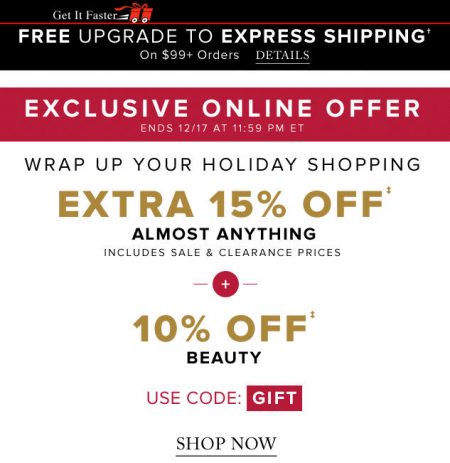This image is an advertisement for a website promoting holiday shopping deals. At the top, the heading "Get Up Faster" is prominently displayed, accompanied by an illustration of a present on wheels with white streaks indicating movement. Below this, a red banner reads "Free Upgrade to Express Shipping," positioned above the text "On $99+ Orders," with a clickable "Details" link.

Further down, there is a white space followed by a red banner announcing an "Exclusive Online Offer" that ends on December 17 at 11:59 PM ET. Beneath this, the text urges viewers to "Wrap Up Your Holiday Shopping" and highlights an "Extra 15% Off Almost Anything," including sale and clearance prices. The "Extra 15% Off" is prominently highlighted in large, gold-colored font.

Positioned centrally, a red circle with a white plus sign indicates an additional "10% Off Beauty," also in gold font. A prompt follows: "Use gift code: GIFT," which is enclosed within a red rectangle. Finally, the advertisement concludes with an underlined "Shop Now" call-to-action.